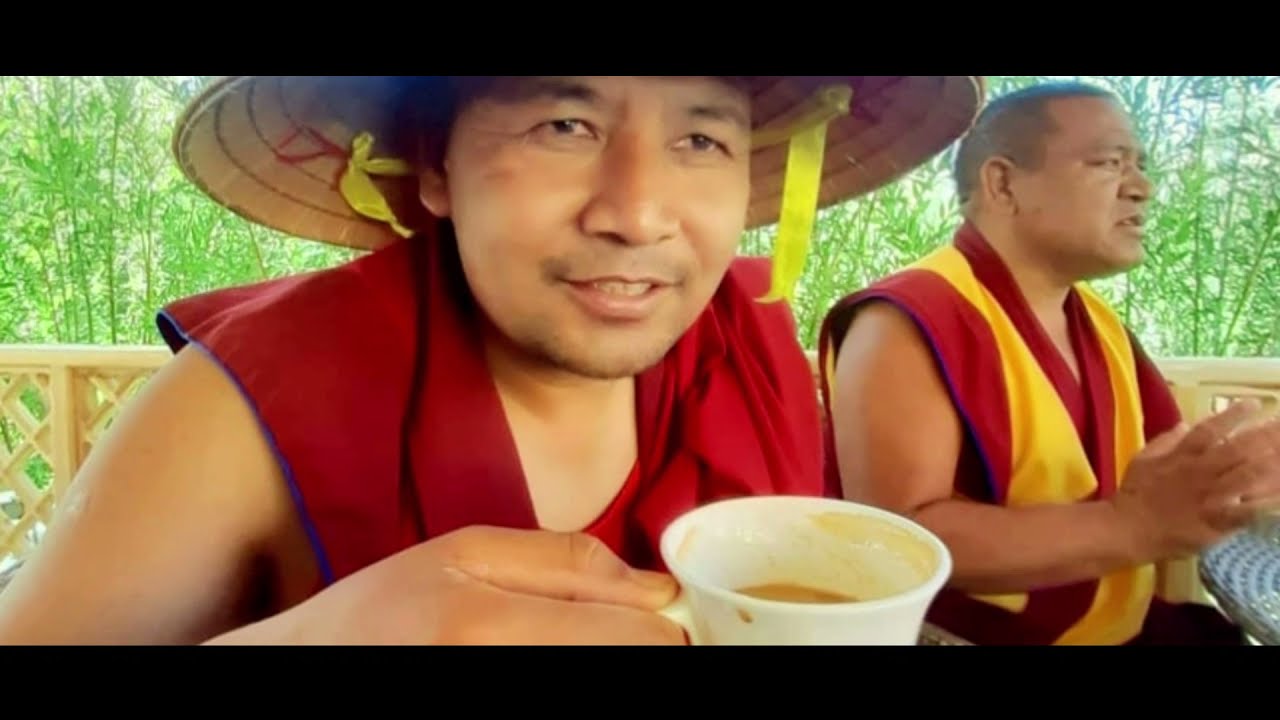The photograph depicts two men with light brown skin, possibly Buddhist monks from Southeast Asia, sitting outdoors on a wooden balcony. Both men are dressed in sleeveless red robes. The man on the left is wearing a wide-brimmed straw hat adorned with white ribbons and is holding a white mug filled with a light brown liquid in his right hand, possibly tea or coffee. The man on the right has short-cropped hair and wears a yellow scarf draped around his neck. He appears to be in mid-conversation, gesturing with his hand. In the background, tall green trees with lush leaves are visible, indicating a partly cloudy sky. The overall color palette of the image includes dominant hues of red, yellow, black, and green. Notably, blue and white striped fabric is seen in the lower right corner, and the image is framed by black bars at the top and bottom.